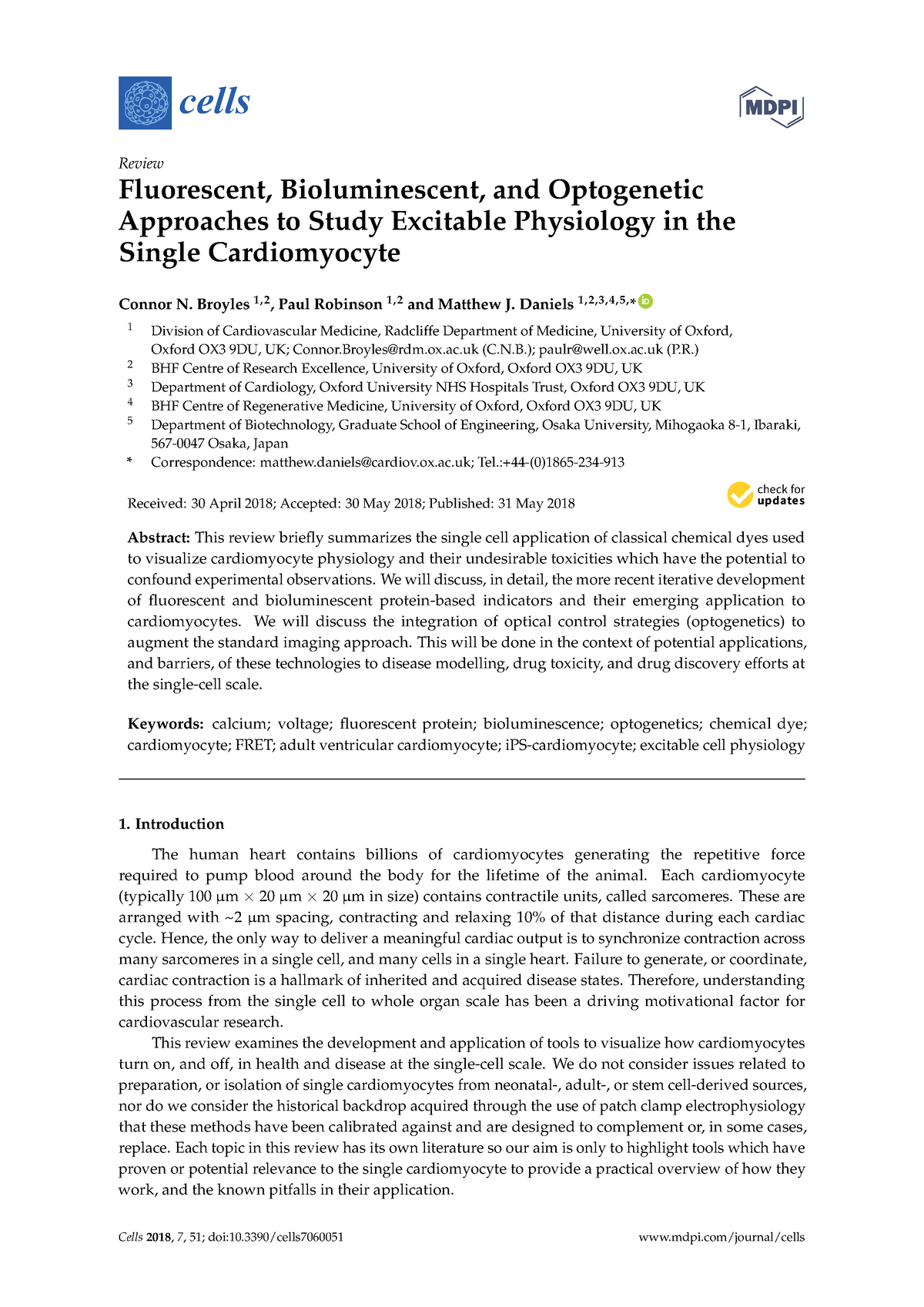This image is from a website that provides detailed information about studying excitable physiology. 

The background of the image is white. In the top left corner, there is a blue square, inside of which is a detailed circular design resembling a cell. The circle is composed of numerous smaller circles, with each smaller circle containing another tiny white circle.

To the right of this design, the acronym "NDPI" is prominently displayed in bold, uppercase letters. The letter "D" slightly tilts up to the left and down to the right, creating a unique visual effect. Just below the "NDPI," in smaller lettering, the word "review" is printed.

Centered on the image, in large, bold black letters, the following text can be read: "Fluorescent, Bioluminescent, and Optogenetic Approaches to Study Excitable Physiology in Single Cardiomyocyte". Below this title, there are three names listed horizontally, followed by information listed vertically next to numbers one through five. 

Near the bottom, there is an eight-line paragraph summarizing the content. Following this summary, keywords are listed in two lines. A black border separates this section from the main text. 

On the left side, just below the black border, the heading "1. Introduction" appears. This is followed by two paragraphs, each about seven lines long, providing further details on the topic.